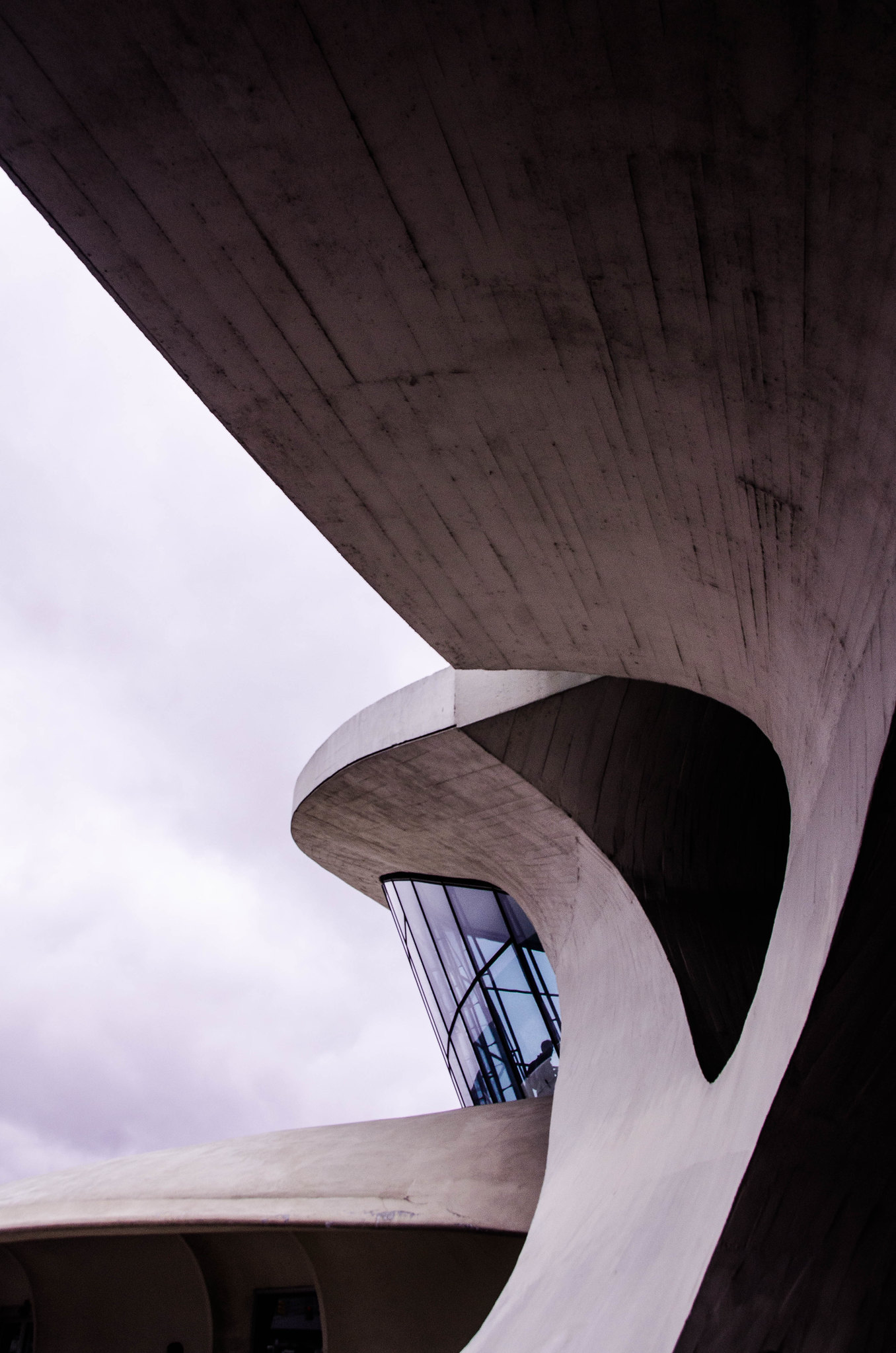A detailed and cleaned-up version of the caption could be:

"Captured from an intriguing angle, this photograph showcases the architectural complexity of a building's side. The structure features an upward swooping design, culminating in an archway at the top. Just below the arch, a glass window juts outward at an angle, through which a person can be seen standing inside. The building appears to have multiple levels, as visible in the section beneath the angled glass, where the roof curves downward before being interrupted by another glass partition. This segment is followed by a more prominent curved roof section closer to the camera. The backdrop is a sky filled with dense white clouds, though the sun is out, casting sufficient light on the building to reveal its fascinating details."